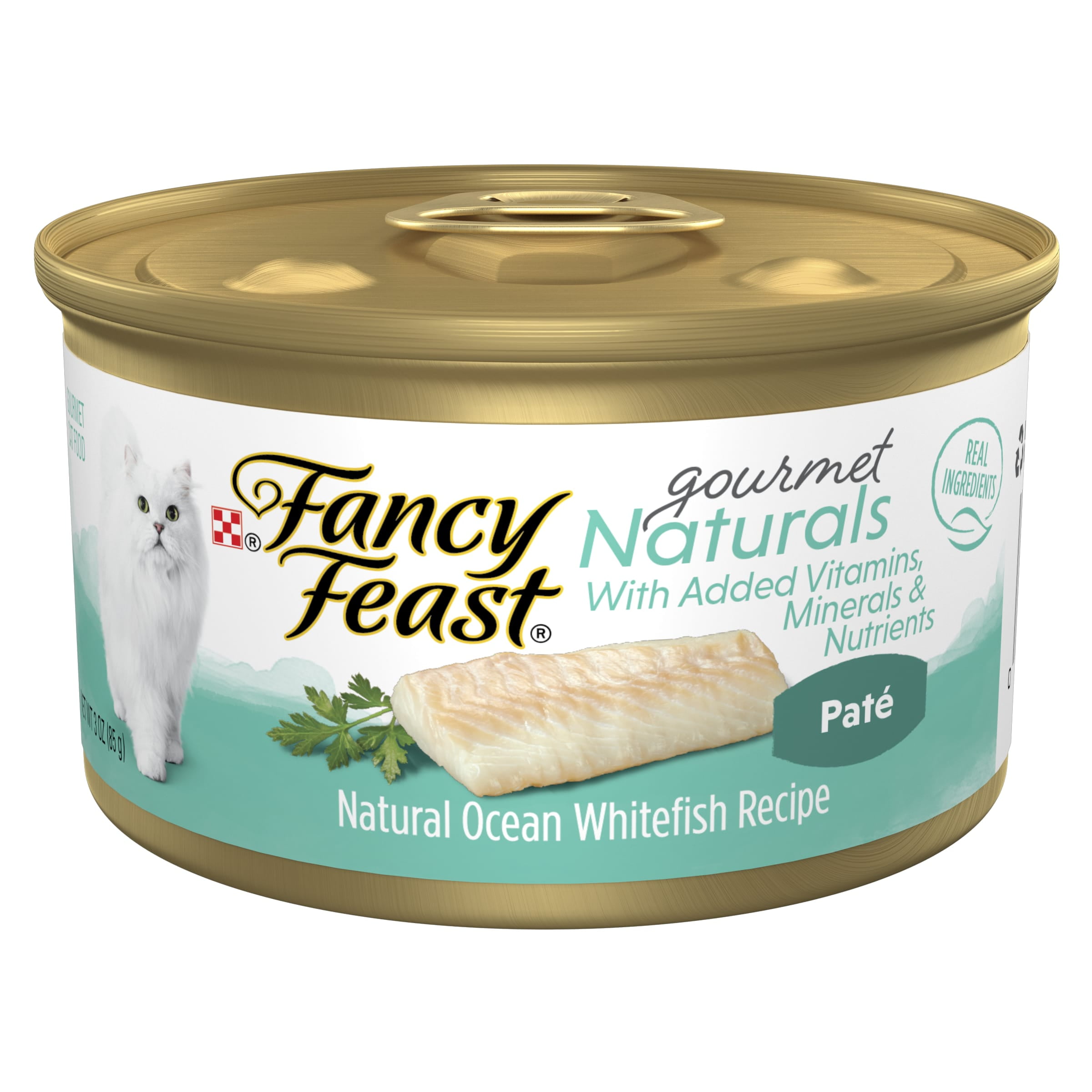The image is a color photograph in a square format, showcasing a can of Fancy Feast Gourmet Naturals cat food with added vitamins and minerals. The gold or brass-colored tin has a labeled center, featuring a white top and aqua bottom. On the label, the red and white Purina checkered logo is positioned on the left, accompanied by a white, long-haired cat with blackish eyes walking towards the camera. The Fancy Feast brand name is written in stacked black script next to the logo. Below it, a piece of natural ocean whitefish with a parsley sprig is prominently displayed. The label also includes text in white on an aqua background reading "Natural Ocean Whitefish Recipe" and is marked with a dark green ellipse containing the word "Pate" in white text. A black script 'Gourmet' is above the text "Naturals" in aqua. The words "Real Ingredients" are positioned in the upper right corner of the can's label. The entire scene is set against a white background, creating a clean and detailed product display.